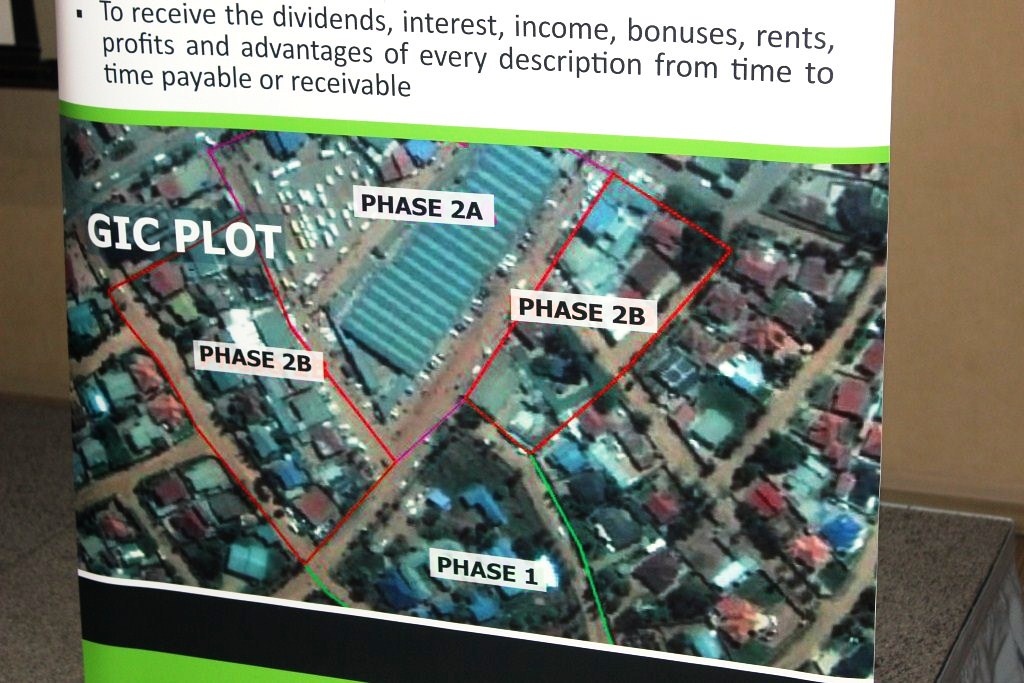The image depicts a top-down view of plots of land, segmented into different phases labeled as Phase 1, Phase 2a, and Phase 2b. A red line highlights the boundaries of these sections. The land is marked as GIC plot and shows various housing units with roofs in different colors (blue, red, and gray) connected by dirt roads. The background setting suggests the image is printed on a piece of vinyl, possibly displayed indoors against a tan wall with a gray carpet visible. The top of the image features a white background with black text stating: "To receive the dividends, interest, income, bonuses, rents, profits, and advantages of every description from time to time payable or receivable." This detailed map, likely part of a new housing initiative, captures the geographical layout and phased division of the development area.